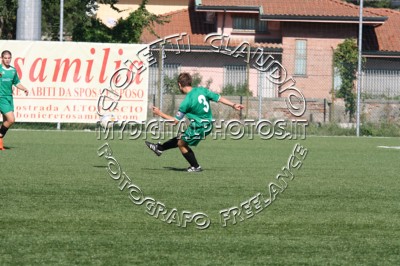In this vibrant, full-color outdoor photograph, two boys in green soccer uniforms, one sporting the number three, are captured mid-play on a lush green soccer pitch. Both boys are wearing matching green jerseys, shorts, long black socks, and soccer shoes. The action scene shows one boy having just kicked a soccer ball, with grassy terrain extending beneath them. Behind them, a girl stands near a large white and red sign that reads "Samila. Abit Da Sponsor."

The picture also features the backdrop of a residential area, with the rear elevation of a brick home prominently visible, characterized by a brown Spanish tile roof. Additional elements in the background include a few flagpoles and tree-covered surroundings, contributing to the overall suburban feel. A watermark in the center of the image reads, "My Digital Photos. Freelance Photography," marking the creator of this sunny day sports snapshot. Dominant colors in the photograph include shades of blue, green, white, brown, black, and beige.